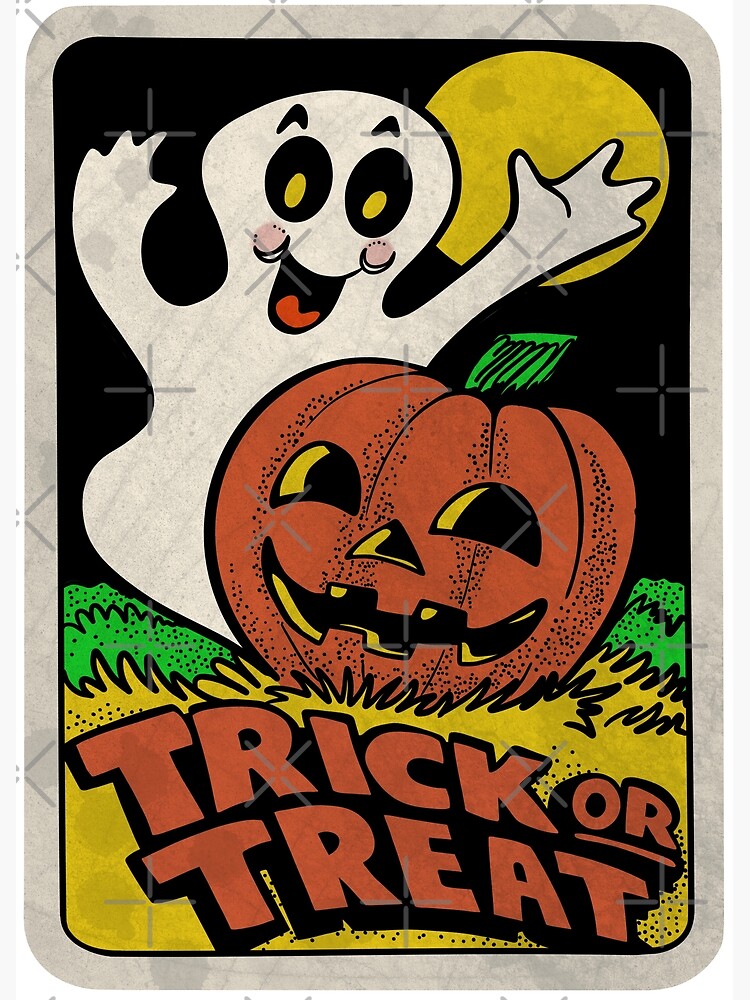The Halloween-themed decorative card, displayed on a white background with a grayish-white border, features a charming illustration. In the foreground, a white ghost with yellow eyes, black pupils, black eyebrows, rosy cheeks, and a red tongue stands upright with arms outstretched, as if about to hug a jolly carved jack-o'-lantern. The pumpkin, adorned with a green stem, slightly leans to the right and sits atop a mix of green grass and yellow hay. Above the ghost, in the top right, a perfectly round yellow moon contrasts against a black sky. The card also includes the phrase "trick-or-treat" in bold, orange block letters on a black background at the bottom. Light gray X's and plus marks watermark the image, giving it a vintage feel and preventing unauthorized copying.